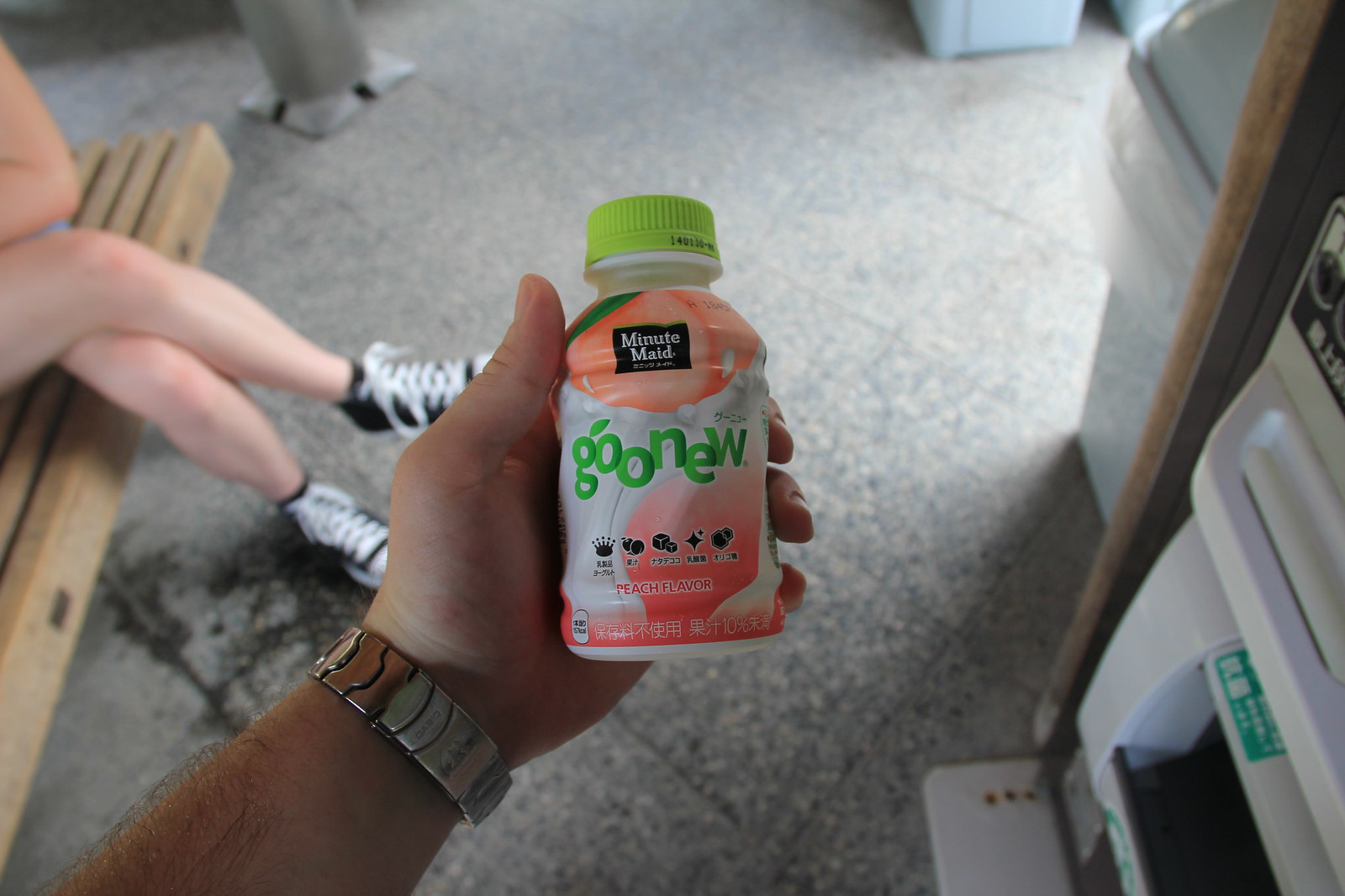The photograph captures a peach-flavored Minute Maid beverage called "Goonoo" (spelled G-O-O-N-E-W), packaged in a small white, green, and pink bottle. The bottle features the brand's name "Minute Maid" and contains both English and Asian script, suggesting it's sold in an Asian market. The drink's label also includes small black images that might indicate texture, nutrition content, or additional flavor details. The photograph is taken at eye level, centered on a muscular, slightly tanned, hairy left arm of a fair-skinned male. His hand, adorned with a thick metal wristwatch, holds the bottle prominently in the frame.

To the left of the image, a woman with a fair complexion sits on a wooden bench, her legs crossed. She sports black Converse Chuck Taylors with white laces. The bench and her attire are clearly visible. On the right side of the image, a variety of items appear, including a possible kitchen appliance and a stove, with gray tile flooring underpinning the scene. A door in the upper right corner lets sunlight filter in, illuminating parts of the background. The overall setting suggests a domestic or informal environment, populated with familiar items and characterized by a casual, everyday ambiance.